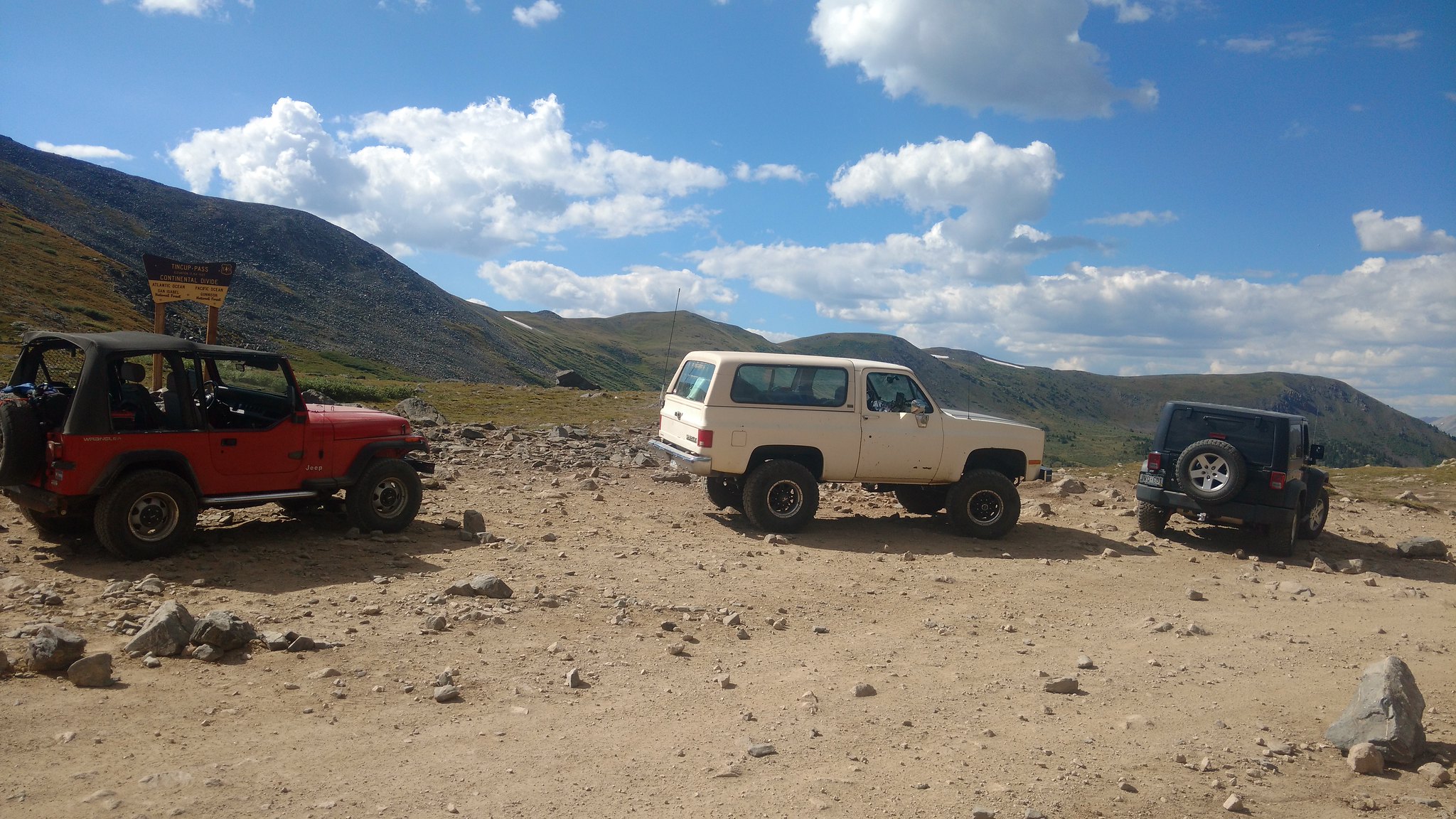The photo captures an outdoor scene featuring three off-road vehicles lined up on a dirt and rocky trail. The leftmost vehicle is a red Jeep Wrangler with a soft top, while the middle vehicle is a white 1980s-style Ford Bronco, reminiscent of the one O.J. Simpson drove. The rightmost vehicle is a newer Jeep, appearing either black or dark green, with the back end facing the camera which makes the exact color indeterminate. This rugged lineup is set against a backdrop of undulating hills covered in green vegetation. Above, a sunny blue sky dotted with a fair number of white clouds adds to the scenic atmosphere. A wooden marker post, akin to those found in national parks or along hiking trails, stands nearby, although its inscription remains unseen. The absence of trees around the parked vehicles emphasizes the barren and natural wilderness of the setting.